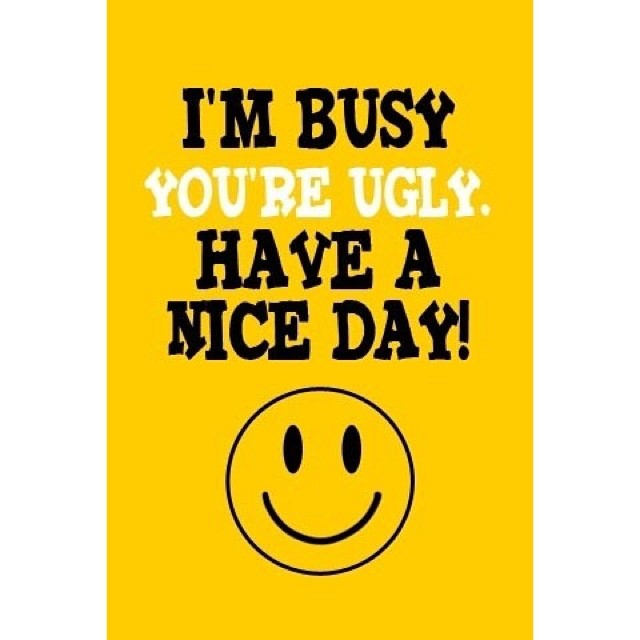The vertically aligned rectangular poster features a bold, solid mustard yellow background without any border. Dominating the top to the center is a string of large, all-caps text conveying a cheeky message. The phrase starts with "I'M BUSY" in thick black letters, followed by "YOU'RE UGLY" in crisp white letters, and ends with "HAVE A NICE DAY!" in black letters again. Beneath this text, centrally placed at the bottom, is a simplistic yet expressive smiley face within a black-outlined circle. The smiley face consists of two elongated black ovals for eyes and a thick upward-curved line for a smile, contributing to its straightforward design. The font of the text appears whimsical with creatively uneven characters, adding a playful yet biting tone to the overall poster.